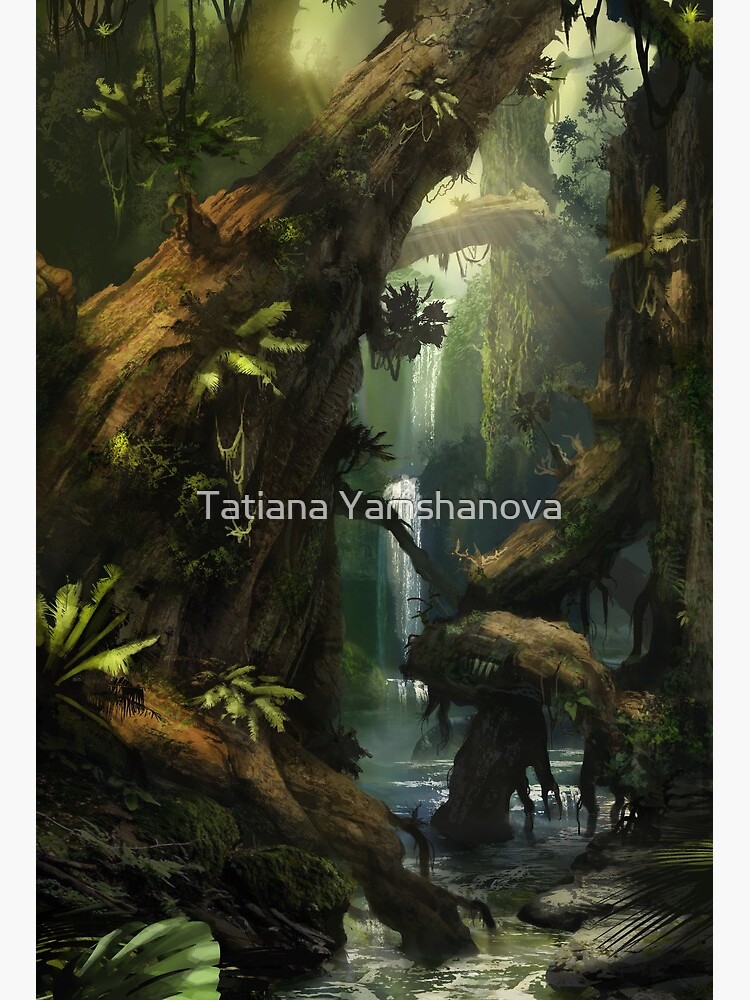This piece is a surreal, detailed digital artwork by Tatiana Yamshinova, depicting a dense and shadowy jungle scene. In the middle of the vertically long composition, the artist’s name is superimposed in semi-transparent white text. The image draws viewers into a lush and intricate landscape with massive, vine-draped tree trunks dominating both the foreground and the background. Beams of sunlight filter through the dense canopy at the top, casting an ethereal glow on the surroundings. Water covers the ground, appearing to flow into a river that starts at the bottom of the artwork. This river transitions into a series of majestic waterfalls about a third of the way up, resembling cascading stairs. Amidst the flora, myriad ferns and fungi grow from the trees, while palm fronds and mossy outcrops add to the jungle's richness. An exceptionally large fallen tree trunk, draped in vines, lies prominently in the scene, contributing to its surreal and slightly menacing atmosphere.